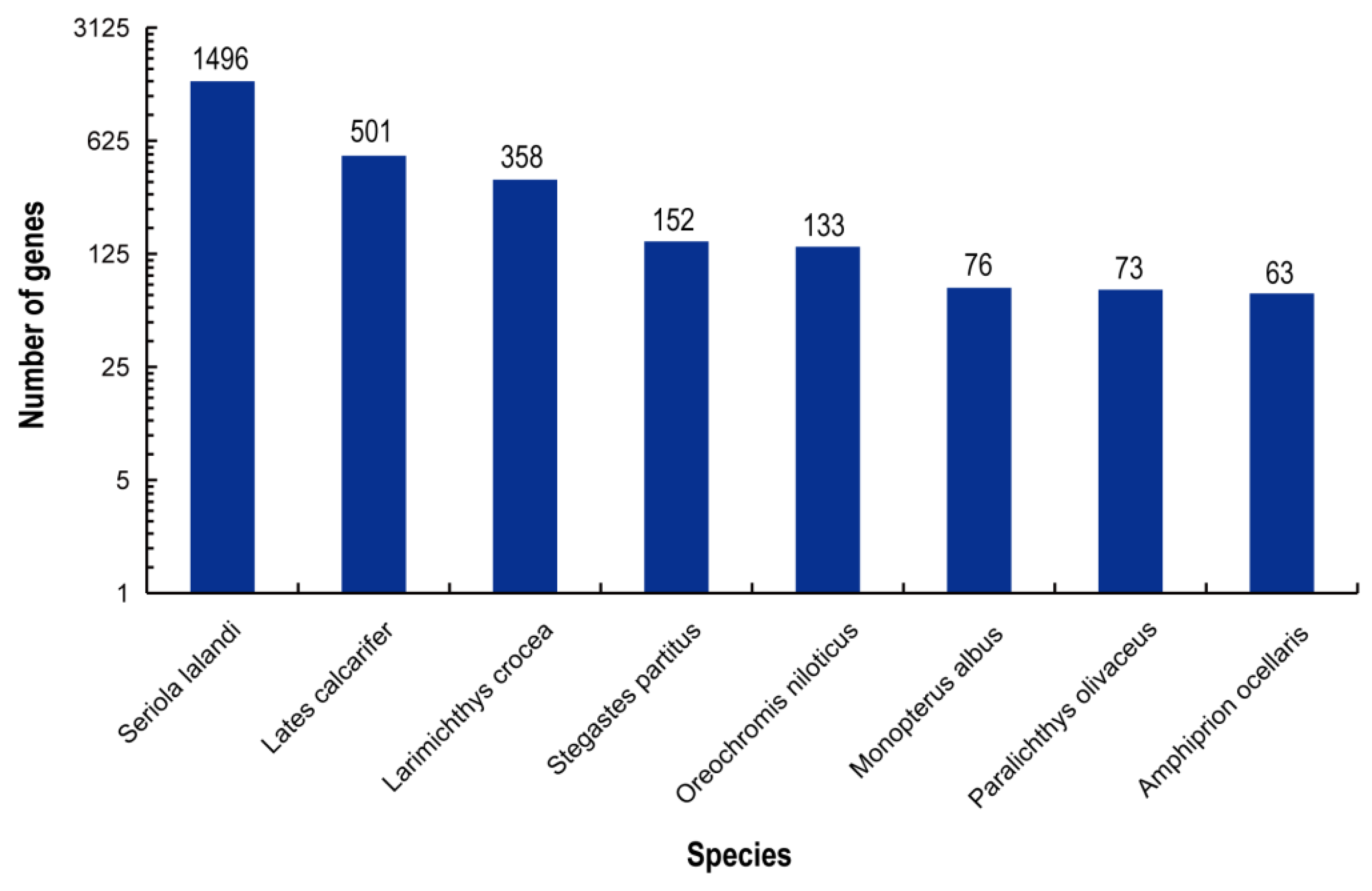The image depicts a horizontally oriented bar graph with a white background, comparing the number of genes across various species. The y-axis, labeled "Number of Genes," scales logarithmically from 1 to 3,125, while the x-axis, labeled "Species," lists eight different species with scientific names. The bars, which are blue, represent gene counts with specific numbers annotated above them. The highest bar signifies Seriola lalandi with 1,496 genes, followed by other species including Lates calcarifer (501 genes), Larvaceis crux (358 genes), and Stegastis partitus (152 genes). The species with the lowest gene counts are Aureochromis nilotiscus (133 genes), Monoterris albis (76 genes), Paralysis olivaxis (73 genes), and Amphiprion ocellaris with the least at 63 genes. Text, numbers, and delineating lines on the graph are colored black, enhancing readability against the plain white background.